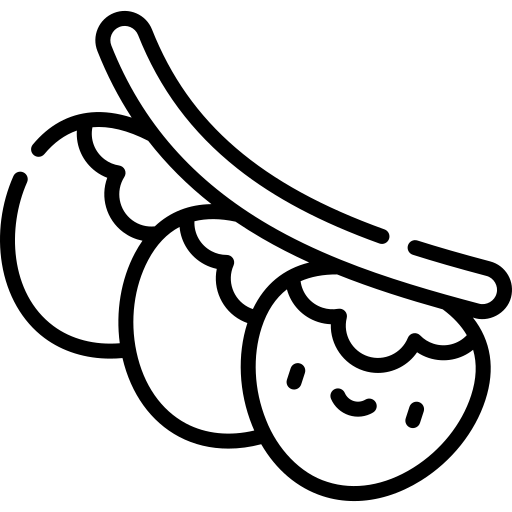The image is a simple, black-and-white digital drawing with minimalistic lines, likely created using few pen strokes. It depicts a curved vine-like stem with three circular shapes attached to it, reminiscent of strawberries. The shapes are positioned along the bottom of the stem, with the one at the bottom-right forefront featuring a happy face consisting of two dots for eyes and a curved line for a smile. Each of these circular shapes has three petal-like leaves. The image has no background or text, reinforcing its straightforward and child-like design, possibly intended for a children's book.